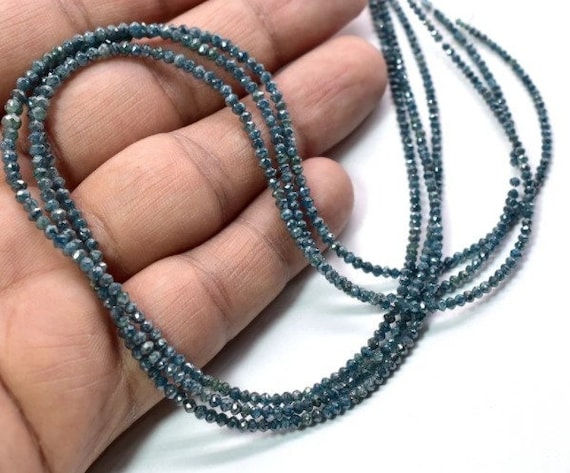The photograph features a close-up view of a person's hand, prominently displaying the pinky, ring, and middle fingers against a pristine white background. The hand, palm up, has visible wrinkles and callouses, indicative of someone who works with their hands. The skin tone is a rich brown, neither white nor black. Resting delicately in the hand are three interwoven strands of beads, creating an intricate figure-eight pattern. The beads are small, slightly shiny, and dark gray-teal in color, resembling polished stones or minerals. The beads are uniformly sized and strung closely together without spacers, giving the necklace a compact and cohesive appearance. There are no other distractions, making the hand and the beaded strands the focal point of the image.